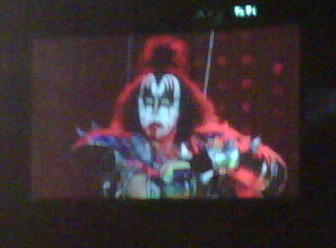This is a blurry photograph, possibly a screenshot from a TV, depicting Gene Simmons from the rock band KISS in his iconic Demon persona. The image has a black border, indicative of a TV screen, with some unreadable white digital text at the top right corner. The center of the image focuses on Gene Simmons, seen from the chest up, against a black and red background reminiscent of stage lighting.

Simmons' face is painted white with exaggerated black eye makeup and what appears to be fake blood dripping from his lips. His hair, predominantly black with a red hue, is styled with a top knot, leaving the rest flowing down. His costume is a black and silver metal outfit adorned with spikes, contributing to his menacing stage presence. The entire scene is bathed in a red hue, likely from the stage lights, enhancing the dramatic and surreal atmosphere of the performance.